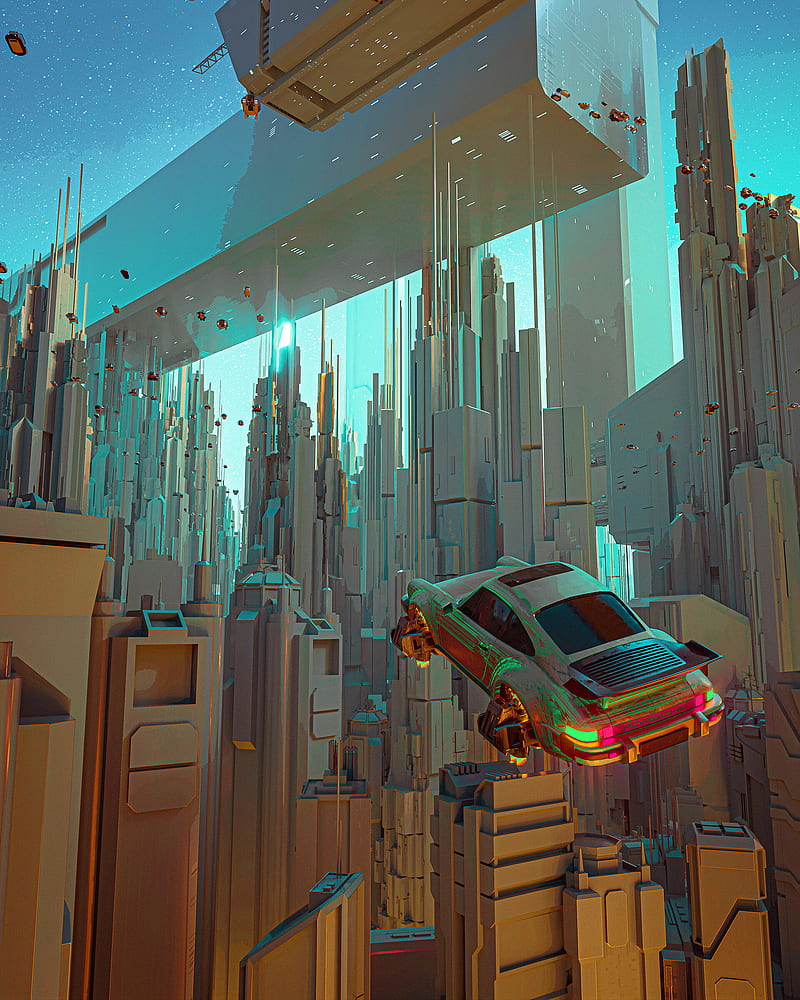The computer-generated image portrays a detailed and vibrant futuristic cityscape, dominated by an array of tall, dense buildings with pointy and jagged tops, lacking windows and rendered in hues of brown and silver. The sky, a blend of aqua blue and light blue, intriguingly displays scattered stars despite the daylight. A large rectangular structure with holes hovers ominously above the city. Numerous flying cars populate the background, creating a sense of bustling activity. Central to the image is a prominently featured flying car, gray with an orange underside, equipped with special wheels for lift-off. The car's metallic body gleams with touches of green, gold, pink, and fuchsia, vividly standing out against the technologically intricate urban landscape. Small red objects float throughout the scene, adding to the surreal and dynamic atmosphere of this futuristic vision.